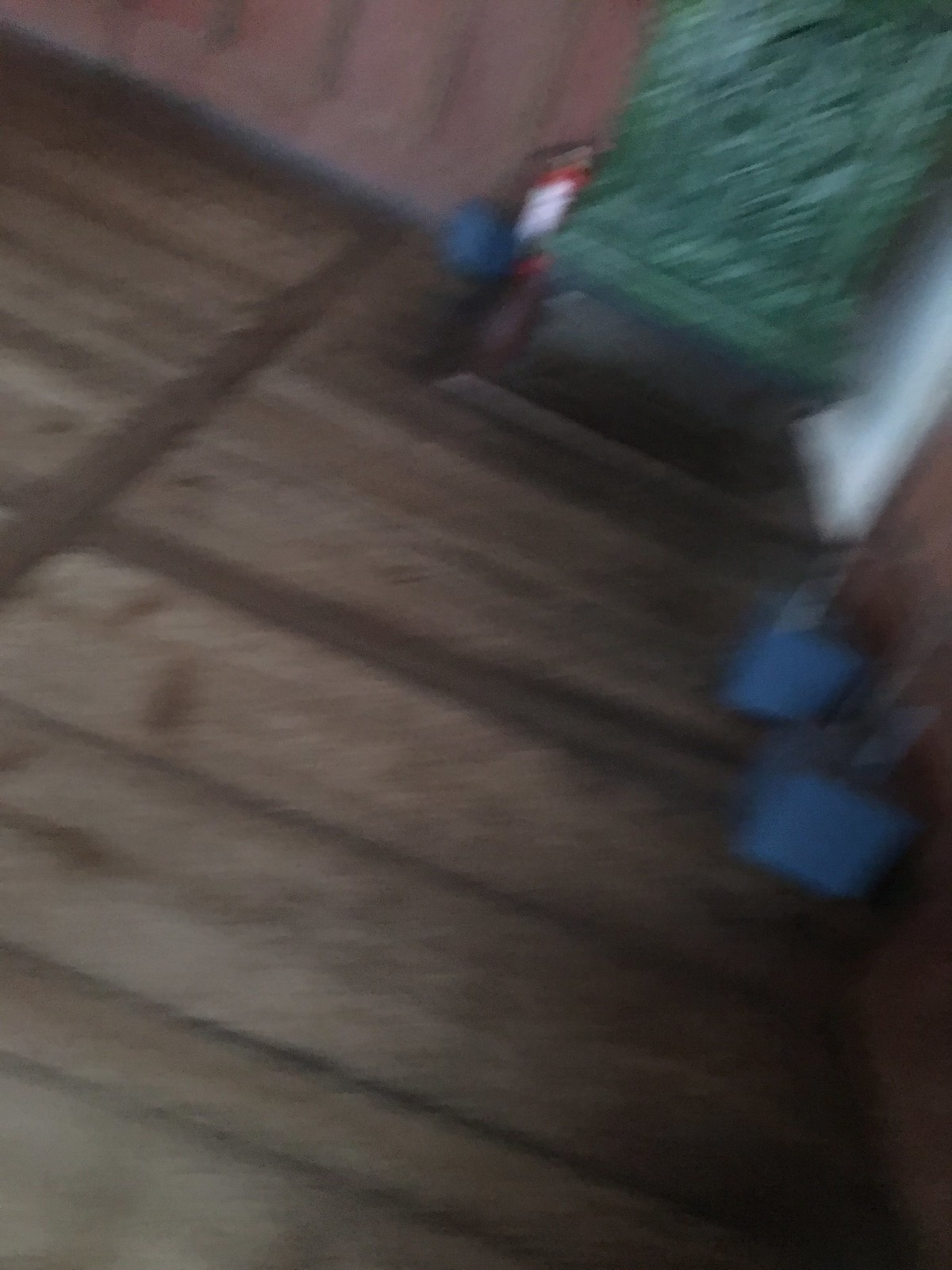The image is a very blurry and out-of-focus photograph of what appears to be an indoor space with a wooden floor. In the upper right corner, there's an opening that seems to lead outdoors to a grassy area. Some blue boxes or planters are situated on the right side of the room, and they appear dark blue in color. A fire extinguisher is visible, though its blurry state makes it hard to distinguish clearly. The foreground floor is wooden with horizontal planks accented by darker stripes. The bottom right corner of the image is dark and shadowy, making it difficult to discern details. Additionally, there is what looks like a white area, possibly a door, on the right side near the blue boxes. Despite the overall blur, these key features can be identified within the scene.